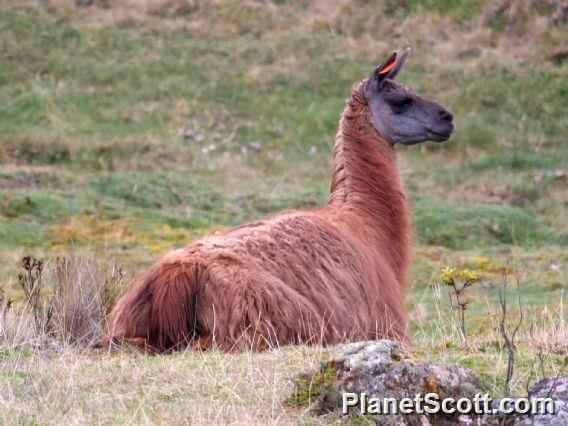In this detailed image hosted on planetscott.com, a copper-colored alpaca with a distinctive grayish-blue face and long neck is seen lounging in a wild, semi-overgrown field. The alpaca is situated in the center of the composition, seated on a patch of grass that appears dry and patchy, interspersed with dirt patches, rocks, and hardy, outdoor plants. The alpaca's body faces the camera while its head turns to the right, presenting its profile with pointed ears and an orange ear tag. The field extends into a grassy hill in the background, displaying various shades of green and brown, indicating areas of straw and wild grasses. The bright, sunny setting illuminates the scene, contributing to the natural yet slightly unkempt appearance of the landscape. The watermark "planetscott.com" is visible in white font with a black outline in the bottom right corner, near a mossy rock from which a few yellow flowers and twigs protrude.